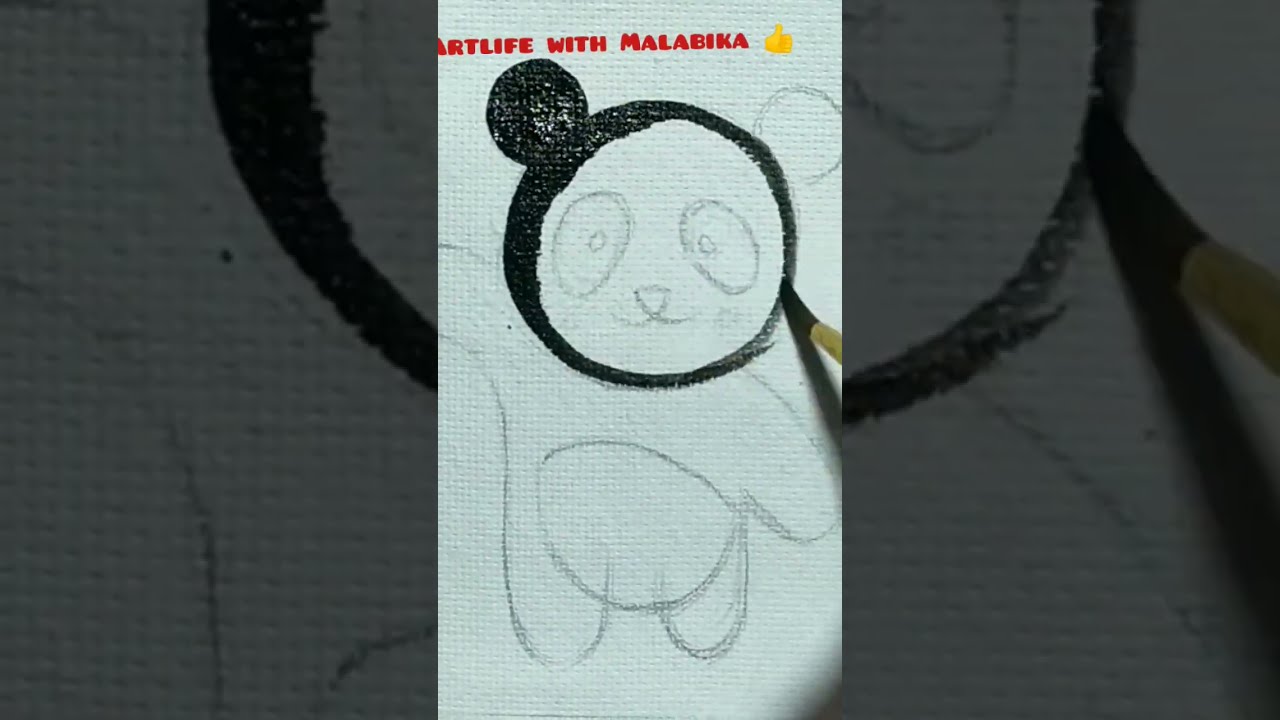The image depicts a partially painted cartoon drawing of a bear, appearing to be a panda based on its coloration. The bear's face is visibly detailed, with white eyes, a smiling mouth, and partially filled-in black features. The left ear is fully painted in black, while the right ear is merely outlined. The artist is in the process of painting, with a brush visible in mid-action, applying black paint to the head area of the bear, which has a circular head shape. The bear's body is sketched with visible outlines of limbs, including two arms and two legs, with its left arm raised and the right arm lowered by its side. Above the bear, in small red font, it reads "Art Life with Malibica" accompanied by a thumbs up emoji. The background of the image is a blown-up, darker version of the bear sketch, adding depth and functioning as a border. This secondary image resembles a magnifying effect, enhancing the focus on the central bear artwork.